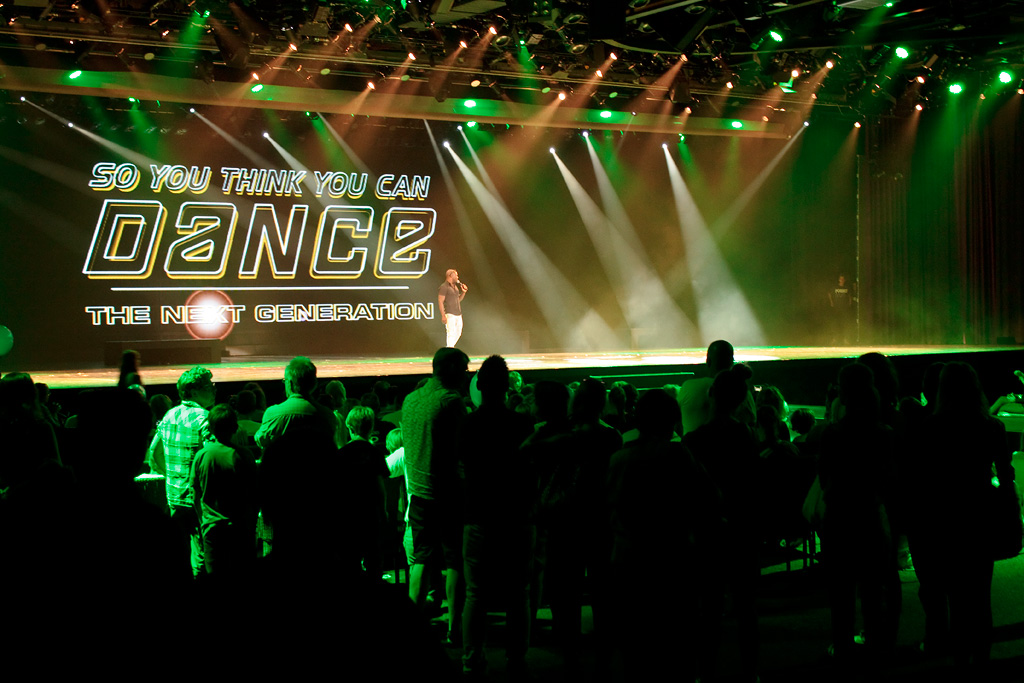In the photograph, an audience anticipates the commencement of a taping for "So You Think You Can Dance: The Next Generation." The room is dimly lit, with the stage illuminated by red, green, and white spotlights that create an atmospheric effect. The backdrop is black, with the show's title, "So You Think You Can Dance? The Next Generation," prominently displayed in large white outline letters. The solitary figure on stage—a man of brown complexion—is dressed in white pants and a dark short-sleeve shirt, holding a microphone as if about to address the audience. The crowd, seen from behind, is bathed in green light, with some members standing and others seated, their silhouettes accentuated by the dim light. The stage is mostly empty, save for the man and a hazy, smoky mist that adds a sense of drama to the scene. Various lights and rigging are visible above, contributing to the intricate stage setup.